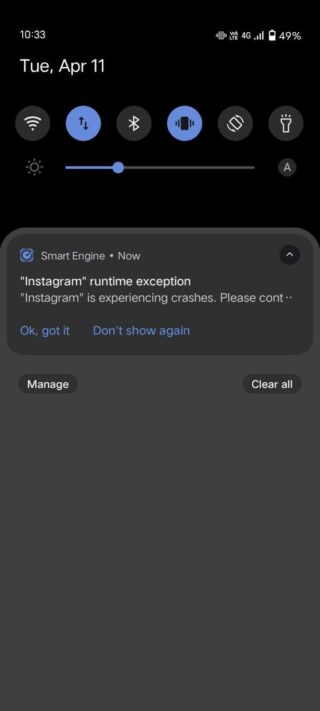A smartphone screenshot with a black background is shown. On the top left, the time is displayed as 10:33, alongside three out of four signal bars indicating 4G connectivity and a battery level at 49%. Below, it mentions the date, Tuesday, April 11th.

The screenshot features a series of icons, starting with a gray Wi-Fi signal icon, followed by a blue icon with an unidentifiable signal symbol, another gray icon displaying the Bluetooth symbol, two more blue icons with indeterminate symbols, and two additional gray icons with unidentified symbols.

Additionally, there is a brightness adjustment icon represented by a circle with lines radiating from it in eight directions. The brightness bar is positioned to the right, showing a blue fill about a quarter of the way, with the remaining portion in gray.

Below this section, the text "smart engine" appears. Underneath, there's a message from Instagram stating, "Instagram Runtime Exception: Instagram is experiencing crashes. Please c-o-n-t..." accompanied by a blue hyperlink with the text "OK Got it."